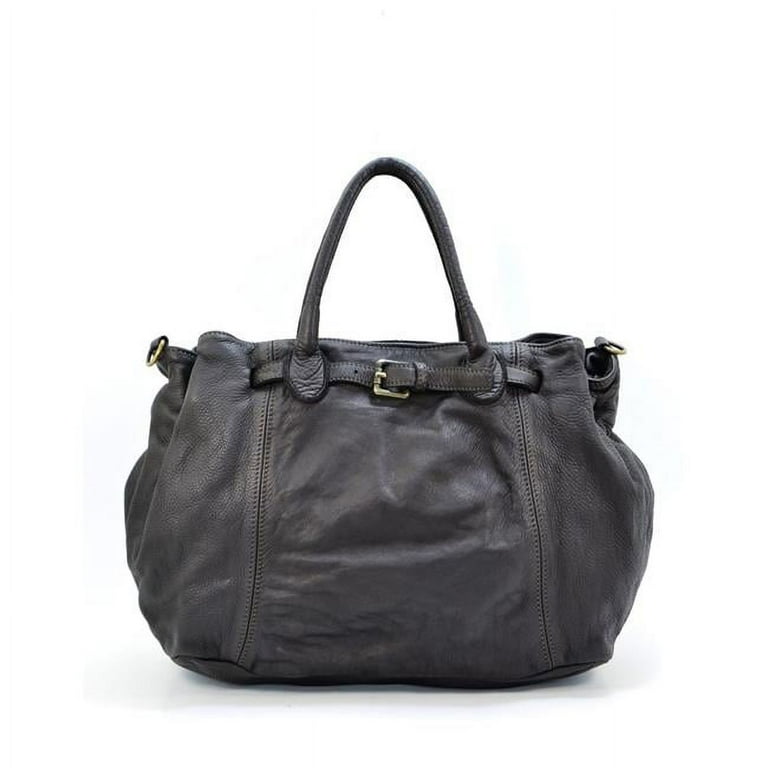The image showcases a medium-sized handbag or purse made of leather material. The bag is predominantly dark grey with subtle hints of dark blue. Noteworthy details include visible stitching along the sides and a belt buckle design positioned beneath the upward-looping handles. Attached to the sides are silver metal circles, likely intended for a larger, detachable strap. The exterior of the handbag also features a white leather section, adding a contrasting element to its overall design.